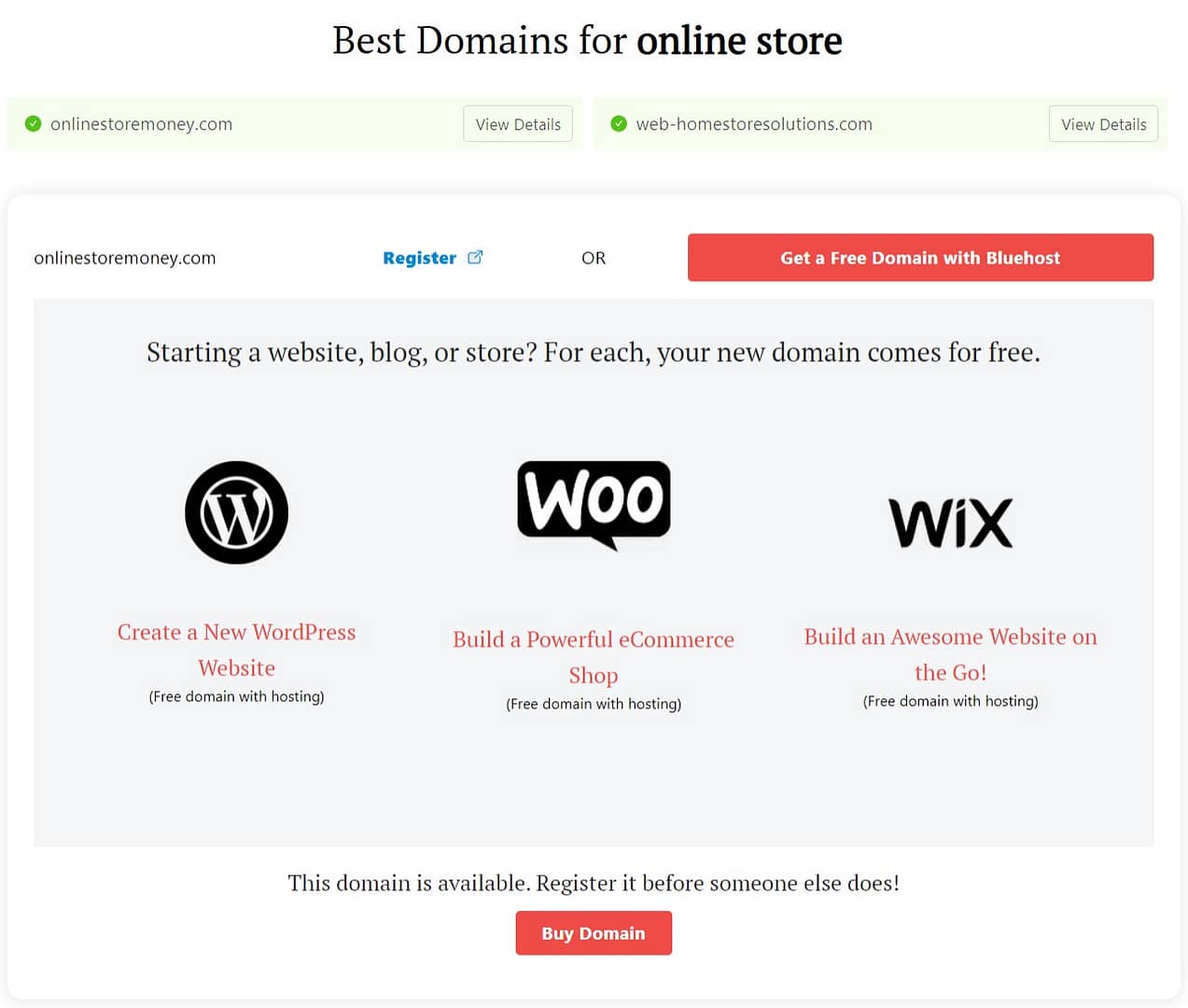This image is a screenshot from an unidentified online source, emphasizing domain registration for online stores. The top portion of the screenshot displays the headline "Best Domains for Online Store," followed by a list of domain names:
- OnlineStoreMoney.com - with an option to "view details."
- Web-HomeStoreSolutions.com - with an option to "view details."
- OnlineStoreMoney.com - with a prompt to "register or get a free domain with Bluehost."

The text below introduces Bluehost, promoting free domain registration with hosting, emphasizing the message: "Starting a website, blog or store? For each, your new domain comes for free. Create a new WordPress website. Free Domain with Hosting."

The image features a series of symbols and logos, including:
- A black circle with a white center containing an uppercase "W."
- A black text bubble with "W-O-O" in white letters.
- Above these, it reiterates the offer: "Build a powerful e-commerce shop. Free Domain with Hosting."
- Another promotional line: "Build an awesome website on the go. Free Domain with Hosting."

Additionally, there is a mention of "WIX" in uppercase letters with the statement "this domain is available" underneath, encouraging users to "Register it before someone else does." This prompt appears in a red rectangle with white lettering that says "Buy Domain."

Notably, the image lacks any photographic elements, people, animals, or plant life. The content strictly comprises text and iconography aimed at domain and hosting services for website creation.